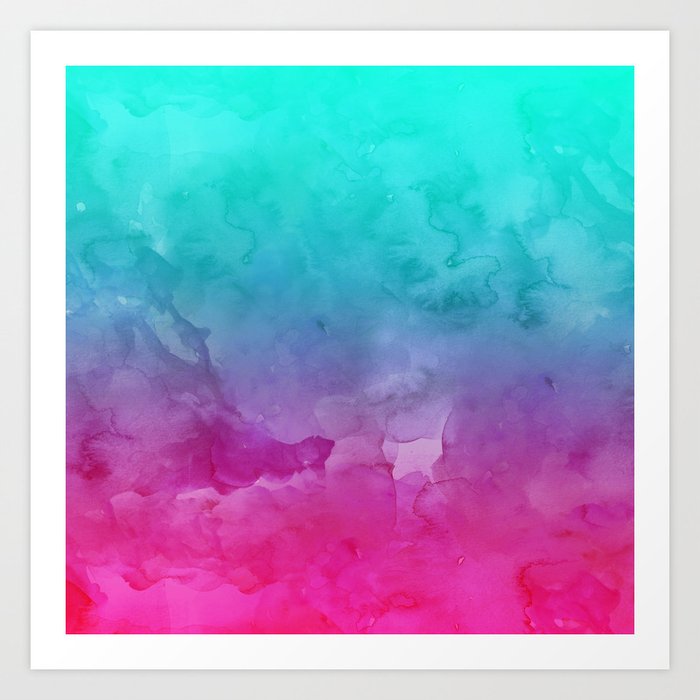The image is an abstract watercolor artwork depicting a smooth gradient of colors flowing from top to bottom. The top of the painting starts with a teal hue, transitioning into lighter blues before merging into purples, and finally culminating in vivid magenta at the bottom. The colors blend seamlessly without distinct lines, evoking the textures of clouds or waves. The artwork features multiple lighter spots, adding subtle complexity to the gentle, flowing pattern. The piece is framed twice: the outer frame is light gray, and inside this is a solid white border. It is displayed on a gray wall, enhancing the delicate and serene aesthetic of the painting.